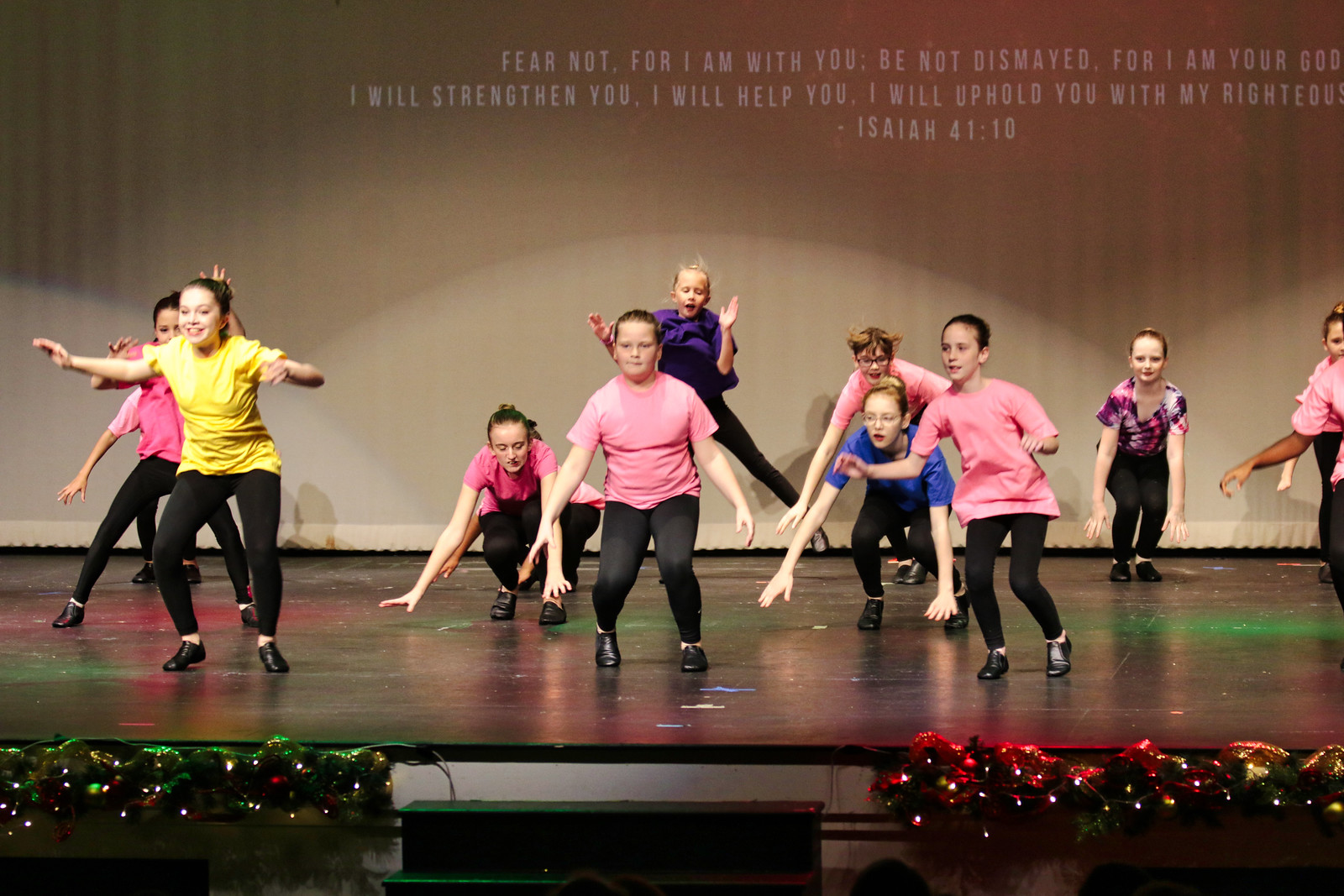On a brightly lit stage framed by green and red decorations, a group of approximately 10 young pre-teen girls performs an enthusiastic dance routine. They are dressed in a variety of brightly colored T-shirts—predominantly pink, yellow, and purple, with one girl sporting a distinctive pink and purple tie-dye shirt. All of them wear black pants and black shoes, and their hair is uniformly tied back in ponytails. The girls strike diverse poses; some are mid-jump with hands raised high, while others crouch, giving the scene a dynamic, lively atmosphere. Behind them, a cream-colored curtain serves as a backdrop, featuring a projected biblical message: "Fear not, for I am with you. Be not dismayed, for I am your God. I will strengthen you. I will help you. I will uphold you with my righteous...," attributed to Isaiah 41:10. The message is partially cropped on the right. Black steps lead up to the stage, adding depth to the lively scene of this youthful performance likely set in a church during a festive season.